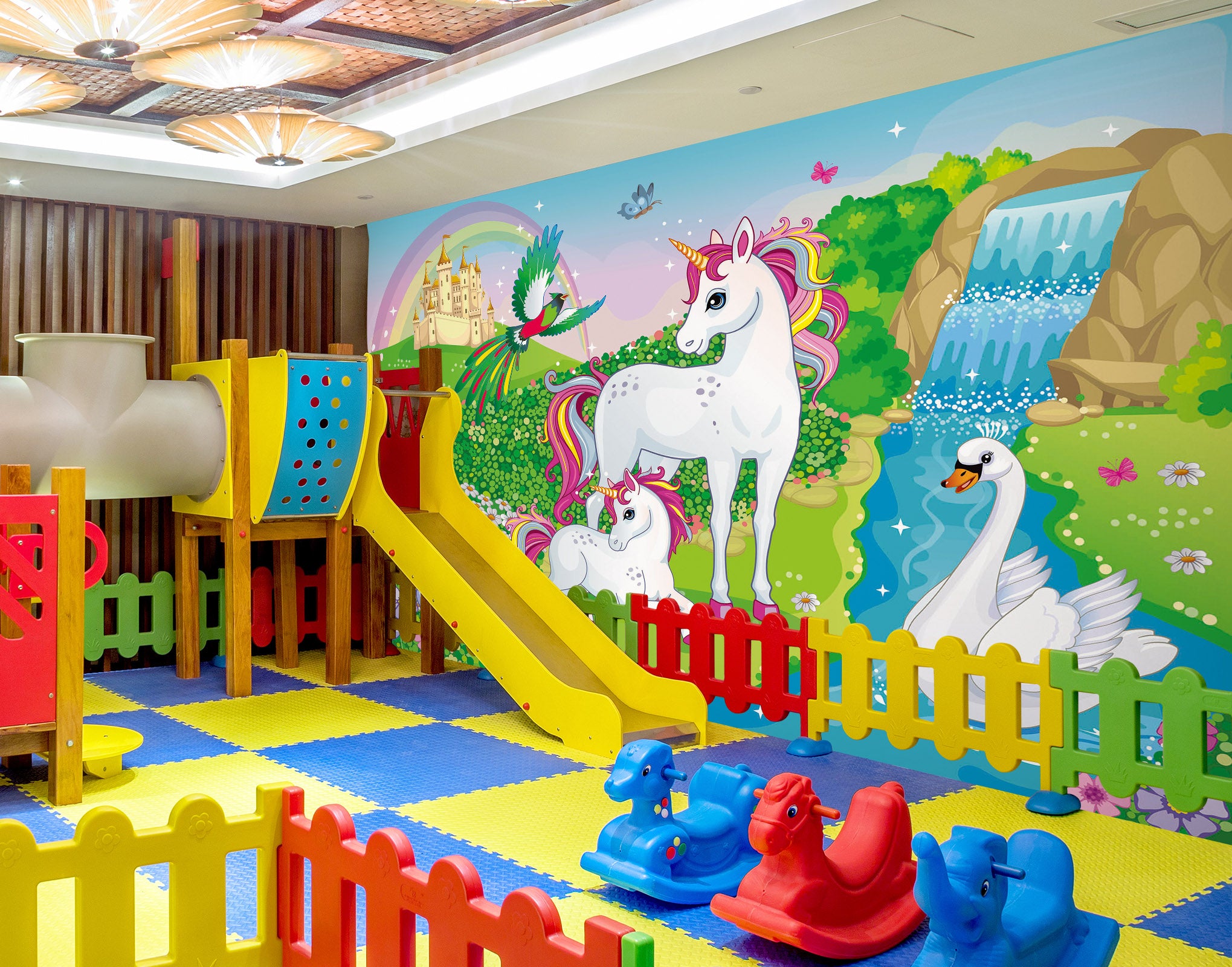The image depicts a vibrant and colorful playroom, possibly in a daycare center. The floor consists of interlocking blue and yellow rubber mat squares, creating a checkered pattern. Surrounding the room is a short, multicolored fence, alternating in green, yellow, and red, effectively enclosing the play area.

Dominating the right side of the image is a large mural featuring an enchanting scene of white unicorns with rainbow-colored manes and yellow horns, a swan gliding on a lake, a massive waterfall cascading down a mountain, and a distant castle with a rainbow arching overhead. Various wildlife, including a butterfly, a bird, and another butterfly, further enhance the magical aesthetic of the mural.

The ceiling is adorned with rounded lights, providing a gentle illumination to the room. In the lower right, there are three small rocking horses, two blue and one red. A yellow slide extends into the room, with metal sides for support, positioned towards the bottom right in front of the fence. Adjacent to the slide is a tube for children to crawl through, which exits the frame on the left side. The corner where the painted wall meets a brown, vertically ridged wall marks the split between the colorful mural and the rest of the room. Overall, the room exudes a lively and whimsical atmosphere, filled with inviting play equipment and captivating artwork.